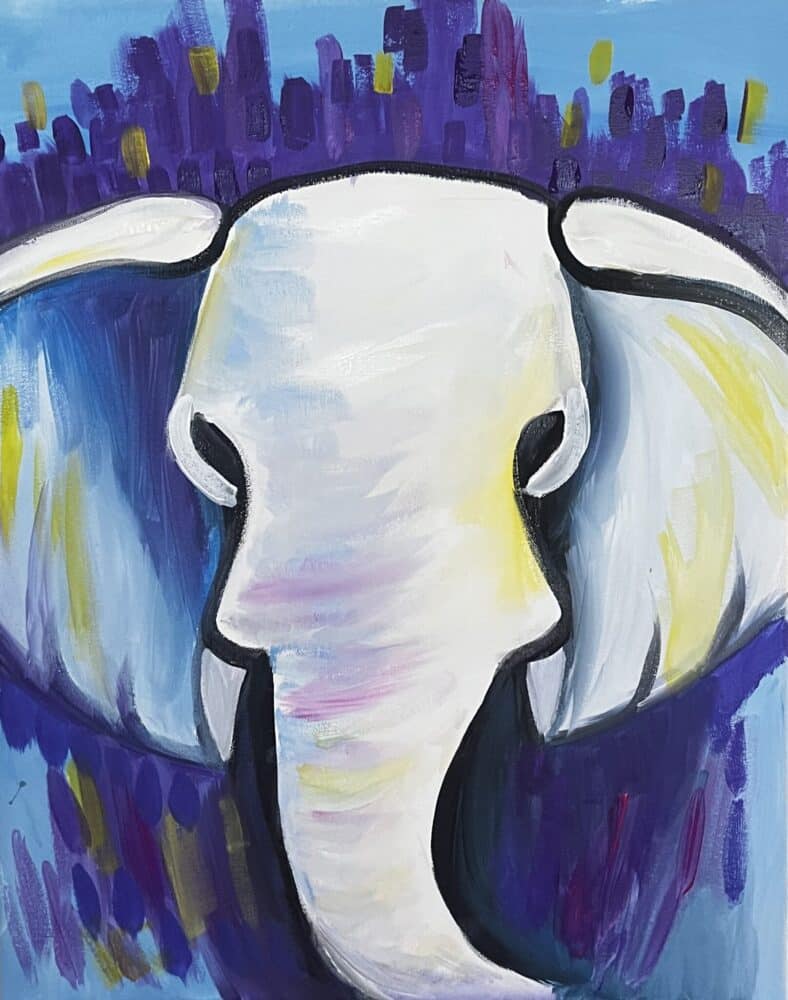This is a vibrant, portrait-oriented painting featuring the head of an elephant, facing the viewer. The main color of the elephant is predominantly gray with dynamic shadow effects incorporating light blue and purple tones. Some parts of the elephant's trunk and ears are highlighted with streaks of yellow, pink, and blue, adding to the overall color complexity. The elephant's left ear, or the ear on the right side of the image, features yellow hues, while the right ear displays more blue and purple shades, possibly mimicking shadows. The elephant’s dark black eyes and the contours of its trunk and ears are defined by heavy black outlines, which give it a striking, almost graphic quality. The trunk swoops downward, curving slightly to the bottom right where the image is cropped. The background is a harmonious blend of light blue with streaks of purple and gold radiating from the top of the elephant's head, extending to the corners. The paint strokes around the head are varied in thickness, some showing drips and edges, contributing to the textured feel of the painting. Overall, the piece creates a captivating and detailed portrayal of the elephant against a richly colored backdrop.